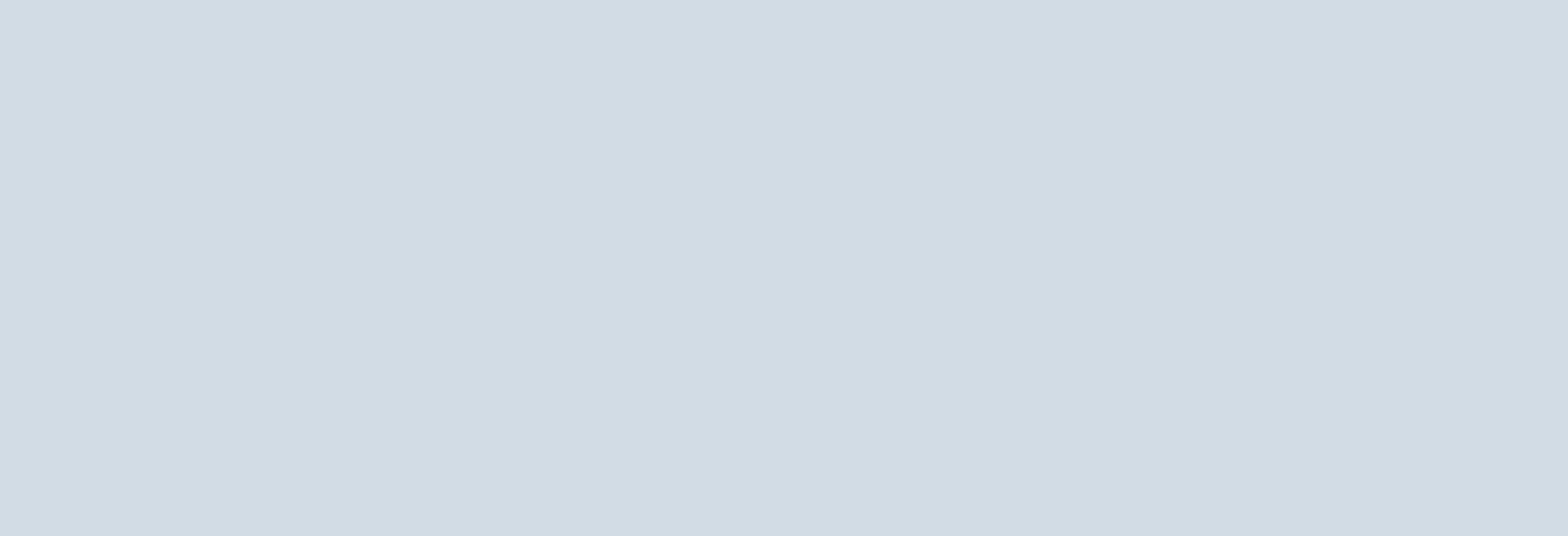Caption: 

An apparent rendering or loading issue on this web page results in a large, featureless grayish-blue rectangle dominating the screen. The rectangle lacks any text or additional details and appears to be a close-up view of the website’s bezel. The image is cut off on all four sides - top, bottom, left, and right - emphasizing the incomplete loading of the page. The composition highlights the technical glitch without offering any further contextual details.